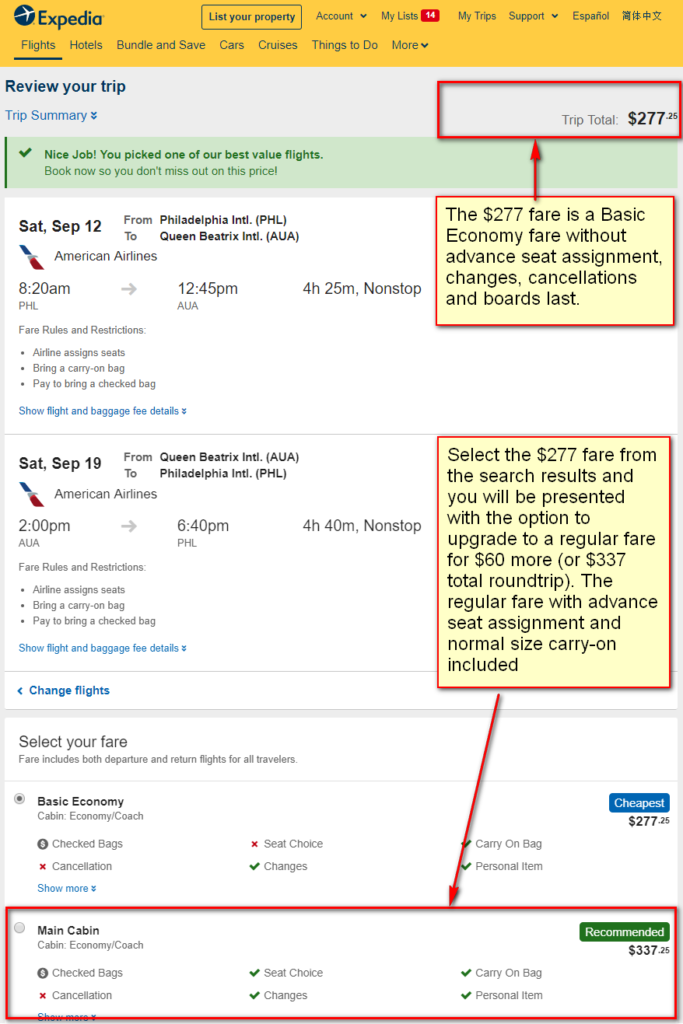A screenshot of the Expedia website is displayed, showcasing details of a travel booking summary on the right side. The page prominently features a section titled "Review of Your Trip." Below this, a breakdown of the trip total is provided, amounting to $2,277.25, enclosed within a red rectangle for emphasis.

Adjacent to this is a yellow box also outlined in red, which is connected to the trip total by an arrow. The yellow box elaborates that the $2,277.25 fare corresponds to a basic economy fare. This fare does not include advanced seating assignments, allows no changes or cancellations, and boards last. 

Further details emerge in another yellow box with a red outline, recommending users to select the $277 fare from the search results. This option provides an upgrade path to a regular fare for an additional $60, totalling $337.25 for a round trip. The regular fare offers advanced seating assignments and includes a standard-sized carry-on.

At the bottom, another box highlighted with an arrow, describes the main cabin economy class benefits. It emphasizes features such as seat selection (indicated with a green check mark), the ability to make changes (green check mark), inclusion of a carry-on bag (green check mark), and a personal item (green check mark). Cancellations, however, are marked with a red X. This option is recommended and totals $337.25.